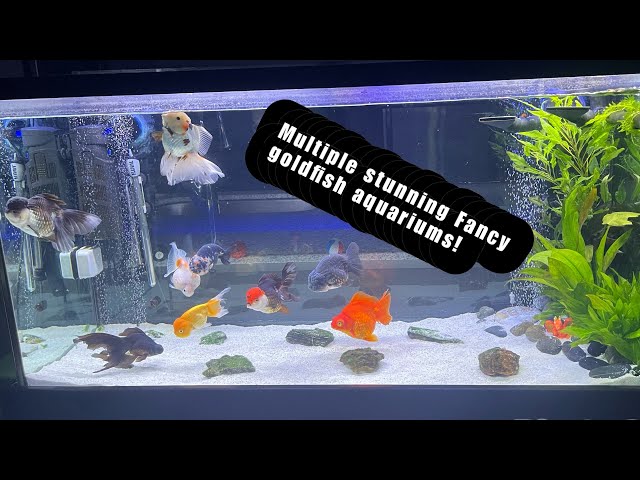The photograph showcases an illuminated aquarium set against a completely dark background, highlighting its vibrant contents. The tank, filled with white sand and a variety of rocks—ranging from shiny small stones to larger rough ones—hosts an array of striking goldfish. Among the dozen fish visible, there are goldfish of various colors, including bright orange, dark gray or black, and multicolored varieties in shades of red, white, and orange. One notable goldfish appears to have bugged-out eyes, and another strikingly resembles a white wedding dress. The fish swim at different levels within the tank, adding a dynamic element to the scene. On the right side of the aquarium, a water filter releases a steady stream of bubbles, partially obscured by a green plant that lends a natural touch to the setup. This plant, along with the reflective surfaces on the left, creates an illusion of a more extensive aquatic environment. Overlaying the tank is a diagonal black banner with white text reading "Multiple stunning fancy goldfish aquariums," accentuated by black stamps making it stand out clearly.